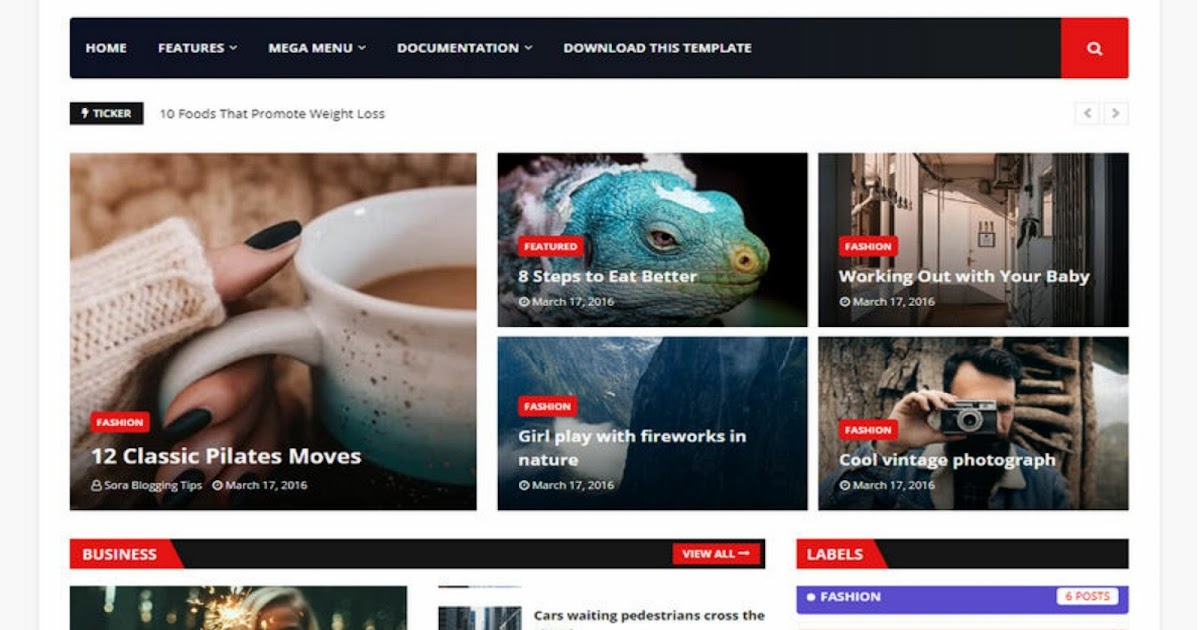The image showcases a clean, organized webpage layout with a black banner at the top. The banner features white lettering with navigation options from left to right: Home, Features, Menu, Mega Menu, Documentation, and Download This Template. On the far right, there is a search button with a red background, white text reading 'Search,' and a magnifying glass icon.

Below the banner, there are five images lined up horizontally:

1. The first image depicts a woman wearing a red and white sweater with black nails, holding a white cup possibly containing coffee or tea. The beverage appears brown. Below this image, "Fashion" is written in red, with "12 Classic Pilates Moves" in smaller white text underneath. At the bottom, the small white text indicates the date "March 17th, 2016."
   
2. The second image features a light blue iguana. In white letters, it reads "8 Steps to Eat Better," with a red background box above it labeled "Featured" in white text. The date "March 17th, 2016" appears beneath.

3. The third image shows a woman, labeled as "Fashion," with white text reading "Working Out with Your Baby." Towards the bottom left, it says "Girl Plays with Fireworks in Nature" in white. The top corner of the image has a red box with the date "March 17th, 2016," and the background features a mountain scene.

4. The fourth image depicts a man with brown hair and a beard, wearing a blue coat with a white, possibly furry, collar. Above the image, "Fashion" is displayed. Below the image, white text reads "Cool Vintage Photograph." Additionally, a black banner on the left side with white text says "Business." A red banner labeled "View All" is to the left.

5. The fifth image is more complex with various banners. The background shows a crowd with the text in white in the middle that reads "Cars Waiting, Pedestrians Cross." Both sides feature navigation labels, with a black banner to the right, fashion blue banner with white lettering.

This descriptive caption captures the precise details and layout of the webpage, ensuring clarity and comprehensiveness.